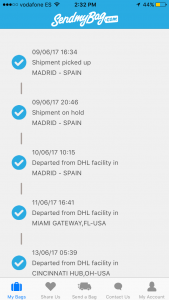A blurry screenshot of someone's phone displays the following details. The top part of the screen is blue, with an unclear word ending in "ONE." Due to the blurriness, it’s difficult to make out the exact word. The time in the middle displays either 2:32 PM or 2:52 PM, and the battery percentage reads 44%, with the battery icon showing it is charging. The background transitions to gray, featuring five blue circles with white checkmarks inside them, indicating the status of a shipment.

1. **Shipment Picked Up**: Location: Madrid, Spain. The date appears to end with "17," likely indicating the year 2017. The time is roughly 16:34.
   
2. **Shipment on Hold**: Location: Madrid, Spain. The time is approximately 20:46.

3. **Departed from DHL Facility**: Location: Madrid, Spain. The unspecified date displays a time of around 10:15.

4. **Departed from DHL Facility**: Location: Miami Gateway, FL, USA. The possible date is November 6th, 2017, and the time is shown as 16:41.

5. **Departed from DHL Facility**: Location: Cincinnati, OH, USA. The probable date is June 13th, 2017, with the time noted as 05:39.

Overall, the screenshot tracks the journey of a shipment from Madrid, Spain, through various locations, including Miami and Cincinnati in the United States.